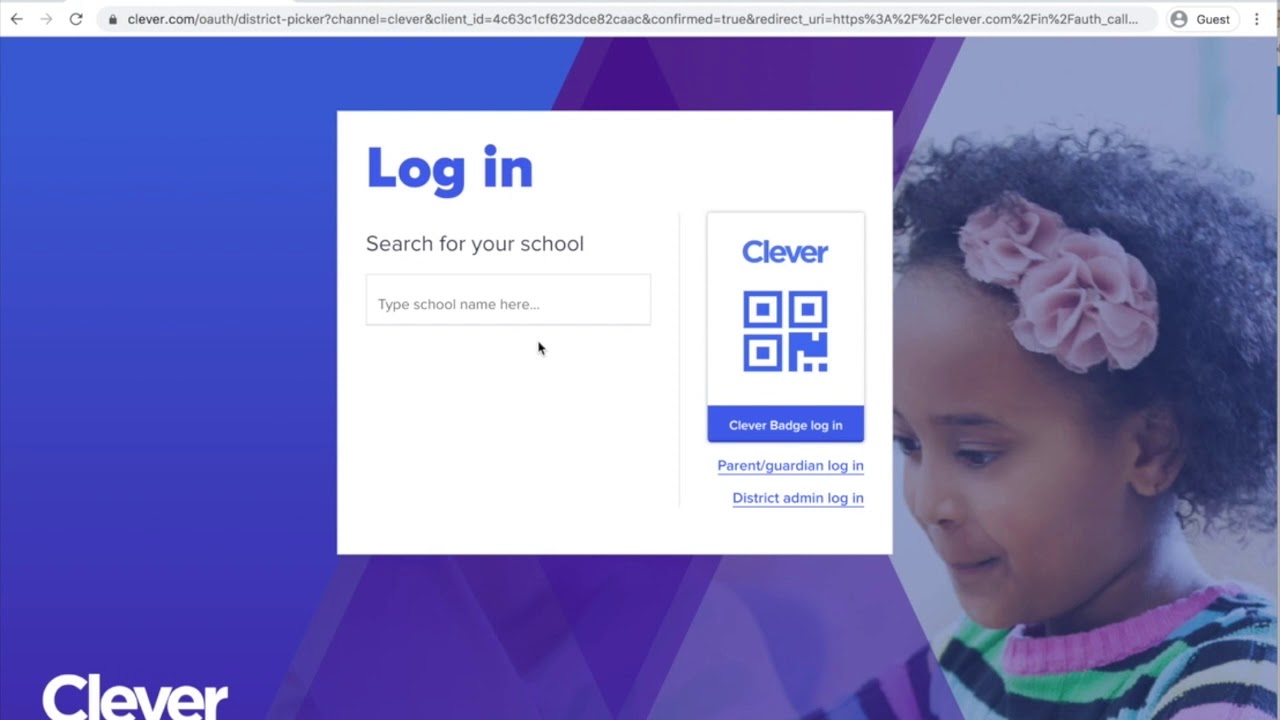The image features a white border along the top, within which several icons are aligned from left to right: a black arrow pointing left in the far-left corner, a gray arrow pointing right, a black refresh button, and a search bar that spans almost the entire width, ending about an inch from the right side. Adjacent to the search bar on the right is a small profile icon and a tab labeled "guest" in black text on a white background.

Centralized in the image is a pop-up tag with a white background, adorned with large, bold blue letters spelling "Login." Beneath this, in black text, reads "Search for your school." Below this instruction is another search bar, highlighted by a black arrow cursor. To the right of the search bar is a QR code with the word "Clever" displayed above it. Following the QR code, there is a blue button labeled "Clever Badge Login." Below this, in underlined blue text, are options for "Parent Guardian Login" and "District of Men Login."

The background of the image transitions through a gradient: starting with blue on the left side, angling downwards to the right where it changes to purple in the center, and finally blending into a pinkish-blue mix along the right side. In the bottom left corner, bold white lettering spells out "Clever."

To the right of these elements is the image of a young Black girl facing left, with her gaze directed slightly downwards. Her pulled-up hair is adorned with two pink flowers, and she wears a subtle smile. Her outfit consists of a striped shirt in green and black with a pink collar.